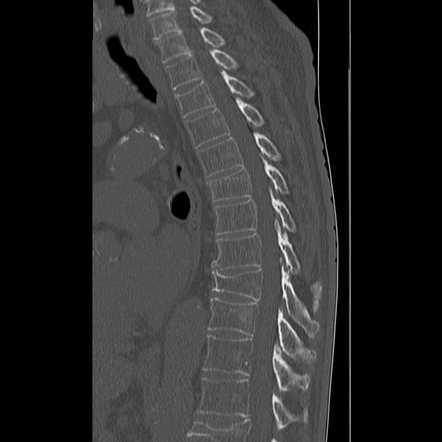This black and white x-ray image predominantly showcases a spine, likely of a human, set against dark borders on the right and left sides. The vertebrae are the central focus, appearing in varying shades of gray to white, with some areas hinting at potential compression. On the left side of the image, there are outlines that might depict internal organs, contributing to the anatomical detail. The contrast between the black undeveloped regions and the highlighted spinal structure provides a clear, albeit non-textual, representation of the internal body.